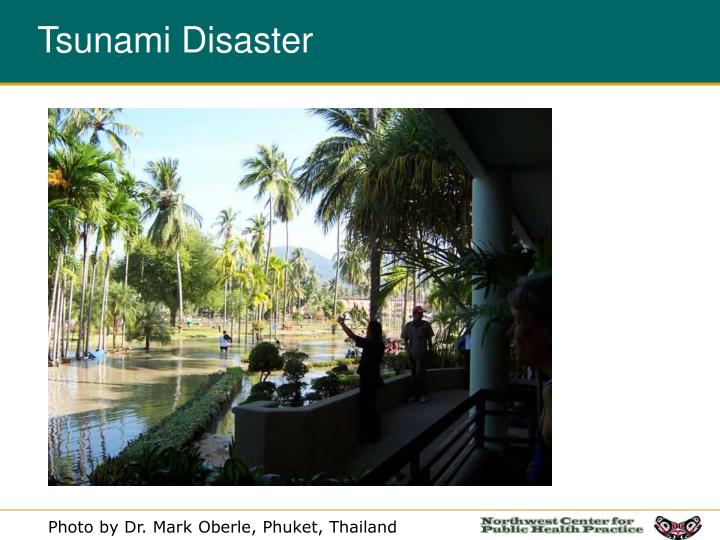The slide features a green banner at the top with left-aligned white text reading "Tsunami Disaster." Below this is a central photograph depicting a flooded tropical area with lush vegetation and many palm trees. The water, which is mostly muddy brown, floods up to a stone wall on the right side of the image, beside a white pillar near a wooden fence. Walking between this fence and wall are two individuals—a man and a woman—with the woman appearing to take pictures and the man looking toward a building. A third person wades through the water, wearing a white shirt. In the background, tall dark green palm trees stretch towards a light blue sky, with the horizon just visible. At the bottom of the slide, text credits the photo to Dr. Mark Oberle, identifying the location as Phuket, Thailand, and includes a logo for the Northwest Center for Public Health Practice. The predominant colors in the image are various shades of brown, green, and blue, highlighting its tropical setting and the impact of the flooding.